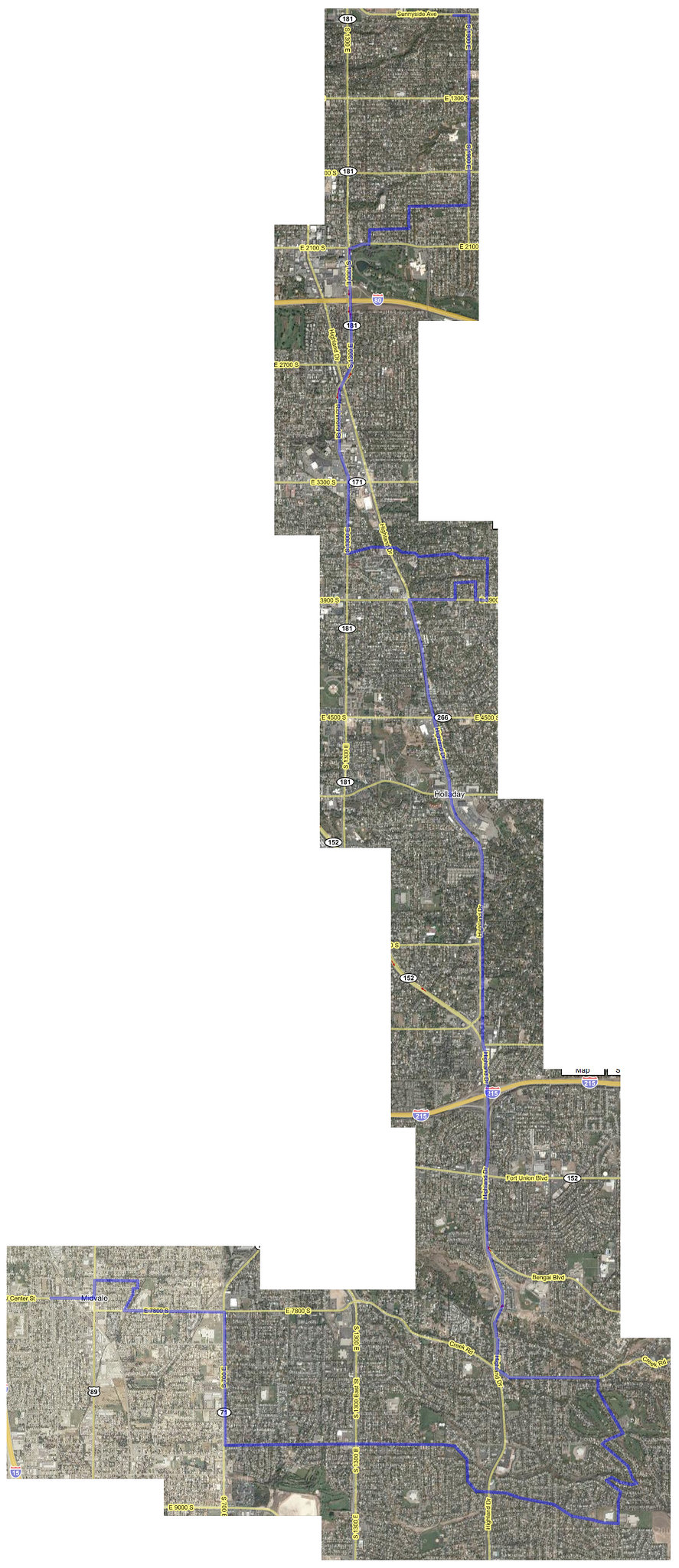This image features a computer-generated patchwork map on a white background. It is composed of eight distinct rectangular segments, which collectively outline a specific route marked in blue. Rather than displaying a full map, only the necessary segments that detail the planned journey are included, creating a mosaic effect. The segments have been meticulously cut and arranged to trace the precise path the traveler will follow, omitting any irrelevant areas. Due to the map's small size, the finer details, such as text and smaller roads, are not discernible, keeping the focus solely on the outlined route.